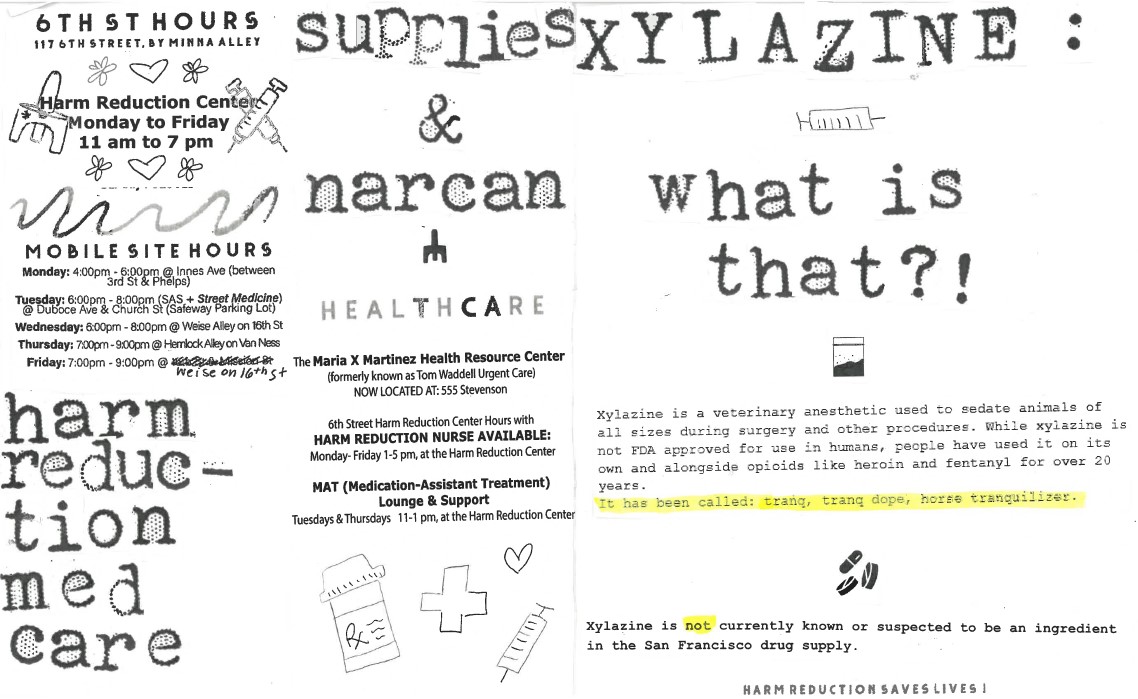The image depicts a detailed flyer for the Maria X. Martinez Health Resource Center, formerly known as Tom Waddell Urgent Care, located at 555 Stevenson. The flyer advertises the Harm Reduction Center, providing various services, including supplies and Narcan, and offering medication-assisted treatment (referred to as "met") lounge and support sessions on Tuesdays and Thursdays from 11 a.m. to 1 p.m. Additionally, the flyer includes important information on 6th Street Harm Reduction Center's hours, noting a harm reduction nurse available from Monday to Friday, 1 p.m. to 4 p.m. Prominently, it also features an explanatory section about xylazine, a veterinary anesthetic used in surgery, which has been utilized alongside opioids like heroin and fentanyl. The flyer has images depicting a pill bottle, a medical cross, and a syringe, and appears to be part of a set of posters commonly found on community boards, providing critical information for those seeking help with drug addiction.